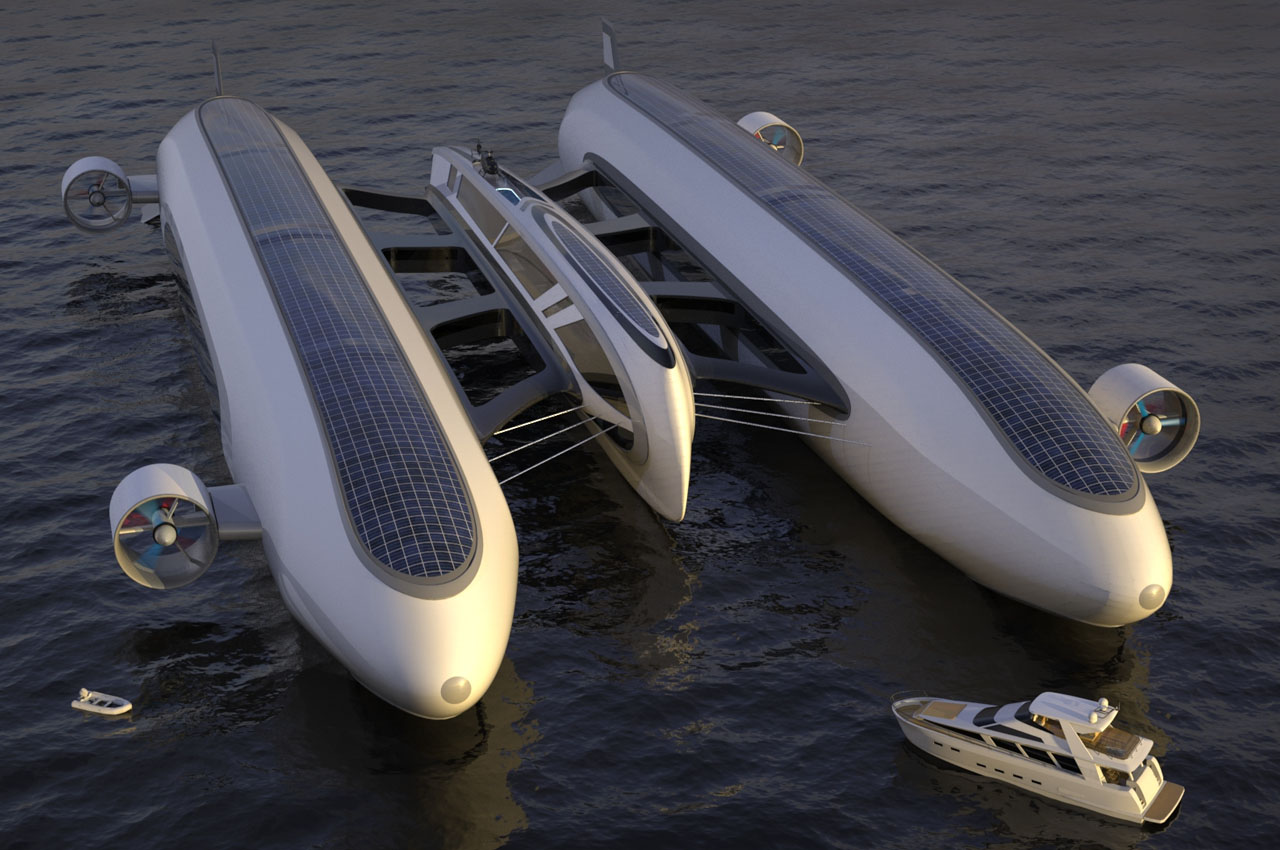This intriguing image showcases a spectacular floating super yacht with a unique and ornate design. The central focus of the image is a massive vessel, resembling a butterfly with a central body and two wing-like structures on either side. This central area appears to house the main living spaces. Docked towards the bottom right is a regular yacht, significantly smaller in comparison – approximately one-tenth the length and one-twentieth the width of the larger vessel.

On either side of the super yacht's central body are two large pods, each nearly double the size of the central section. These pods are equipped with black solar panels on top, providing a sustainable energy source. The pods are white, complemented by black connecting struts and supported by four main beams on either side. To either side of these pods, large propellers are visible, designed to propel the yacht through the water. Towards the rear of the yacht, a sleek black helicopter is perched, adding to the vessel’s opulent features.

Overall, this super yacht exudes luxury and innovation, seamlessly blending striking design elements with advanced technology.